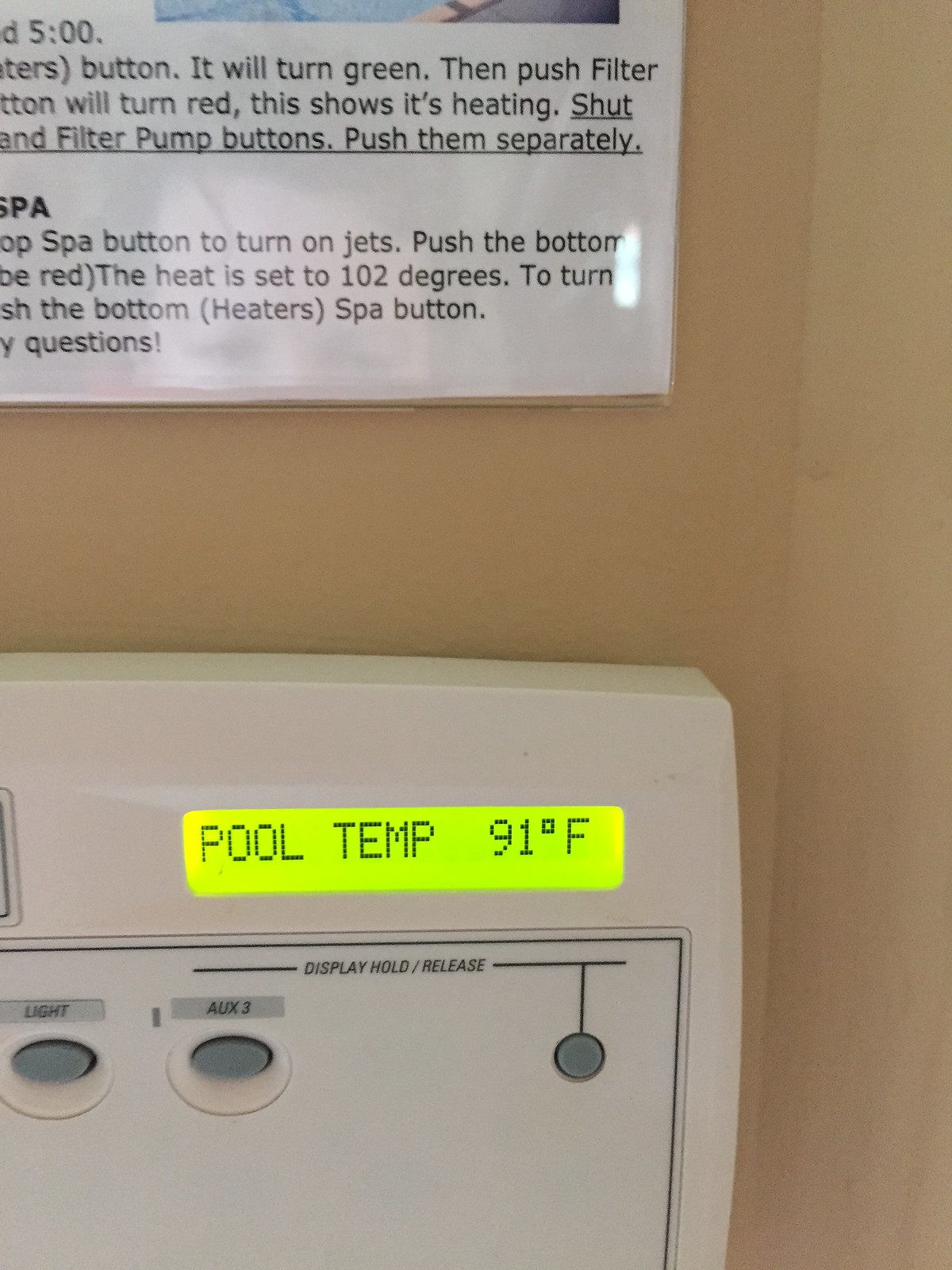This is a detailed photograph capturing a section of a beige or parchment-colored wall, where the corner of the wall turns to the right. Prominently featured on the upper left is a white sheet of paper encased in clear plastic, with only about a quarter of it visible. The sheet contains black print and is mounted securely to the wall. Below this, in the left-central to lower portion of the image, there is a substantial beige plastic thermostat.

The thermostat features a horizontally aligned rectangular screen at its top, lit up in a greenish-yellow hue. The digital display on the screen reads "Pool Temp, 91 degrees Fahrenheit" in dotted text. Situated below the screen, two oval-shaped gray buttons are arranged horizontally. The left button is labeled "Light," and the right is labeled "Auxiliary 3." Above these buttons, a label reads "Display Hold/Release." To the right of the oval buttons, there is a solitary round gray button. The image effectively captures the functional and instructional elements present on the wall.